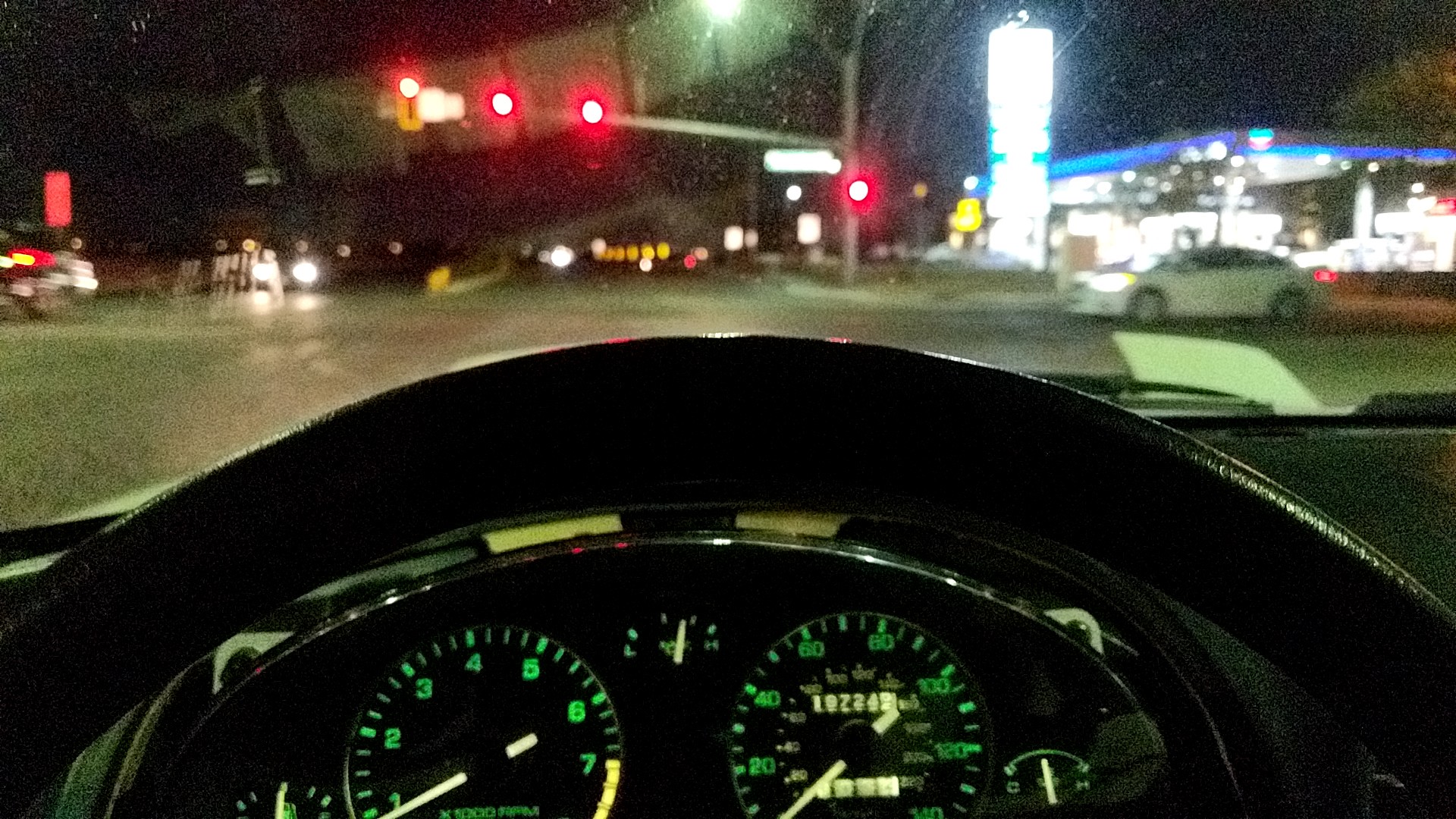This horizontally oriented photograph captures the interior of a stationary vehicle, prominently displaying the dark outline of the steering wheel and the illuminated dash panel. The gauges and controls are clearly visible, with neon green backlit numbers and a white-lit mileage area, although the details appear slightly blurred. The windshield is slightly fogged up or dirty, with visible streaks. Through the windshield, you can see the street at a busy intersection, marked by a large traffic light pole with four lights, three red on a crossbar and one yellow light for a left-hand turn lane. The vehicle is at a stoplight, indicated by the red lights ahead. On the right-hand side of the vehicle, a white car is either waiting or passing through the intersection. The brightly lit gas station directly ahead adds to the scene's illumination. The background reveals additional road signs, yellow headlights, red tail lights of other cars, and a central barrier dividing the street. The overall scene is slightly blurred but vividly conveys the bustling nighttime city environment.